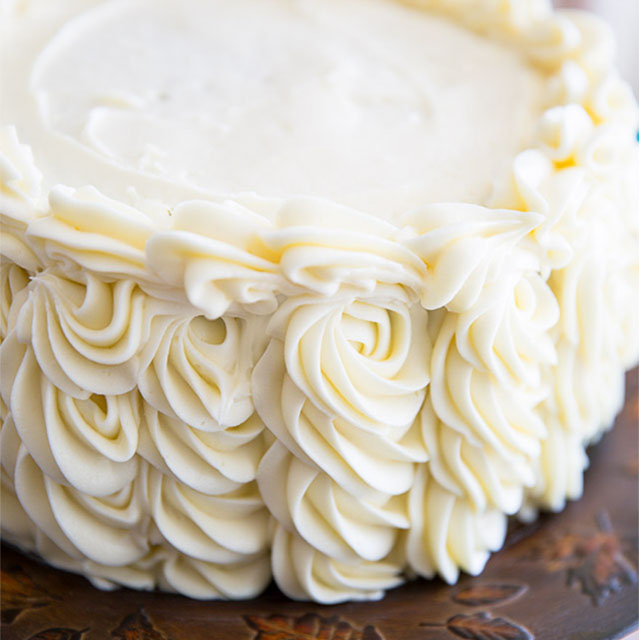The image depicts a close-up photograph of a small, cylindrical confectionary, likely a cake or a fancy cupcake, adorned with an abundance of white frosting. The frosting is meticulously piped into intricate flower shapes, which are bunched together in vertical columns running down the sides and around the top perimeter. The top of the cake features a smooth layer of icing, slightly curved due to the smoothing tool used. The cake is set on an elegant, dark brown plate decorated with engraved leaves in brown and yellow hues, enhancing the overall aesthetic of the presentation. The detailed craftsmanship of the frosting and the ornate plate suggest a dessert designed for a refined experience.